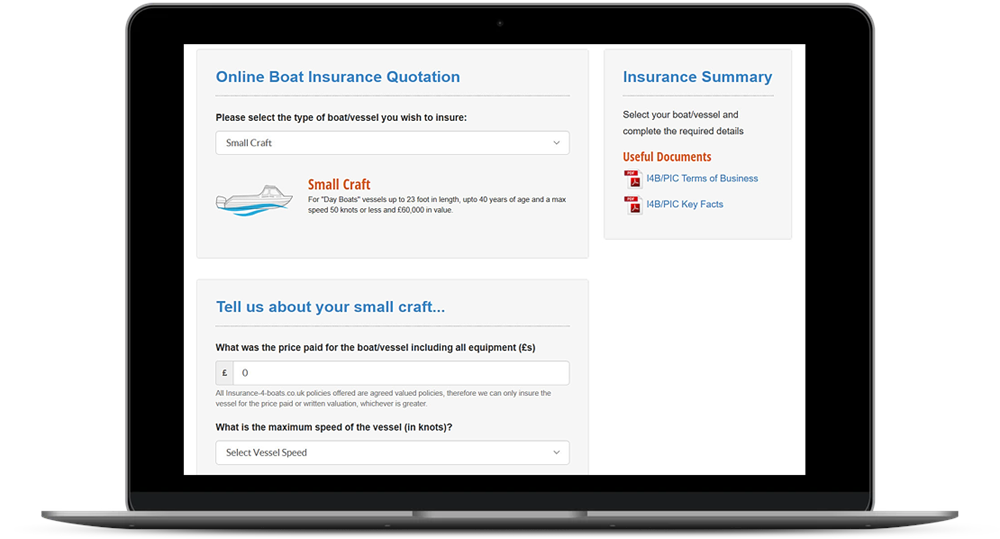The image features a laptop displaying a web page dedicated to obtaining online boat insurance quotations. The laptop is open, revealing the screen with clarity. At the top of the web page, there is a heading that reads "Online Boat Insurance Quotation." Directly below, a prompt instructs the user to select the type of boat they wish to insure from a dropdown menu, with "Small Craft" currently selected. 

The webpage defines "Small Craft" as day boats up to 23 feet in length, with an age of up to 40 years, a maximum speed of 15 knots or less, and a value of $60,000 or £60,000. Underneath this, there is a section labeled "Tell us about your small craft," which asks for the price paid for the boat, including all equipment. There is an entry box provided for inputting this information.

Additionally, a note states that all policies offered by the website (boats.co.uk) are agreed value policies, insuring the vessel for the price paid or the written valuation, whichever is higher. Below this, the user is prompted to enter the maximum speed of the vessel in knots via a dropdown menu. On the right side of the screen, an insurance summary is visible, providing a concise overview of the entered details for the quotation process.